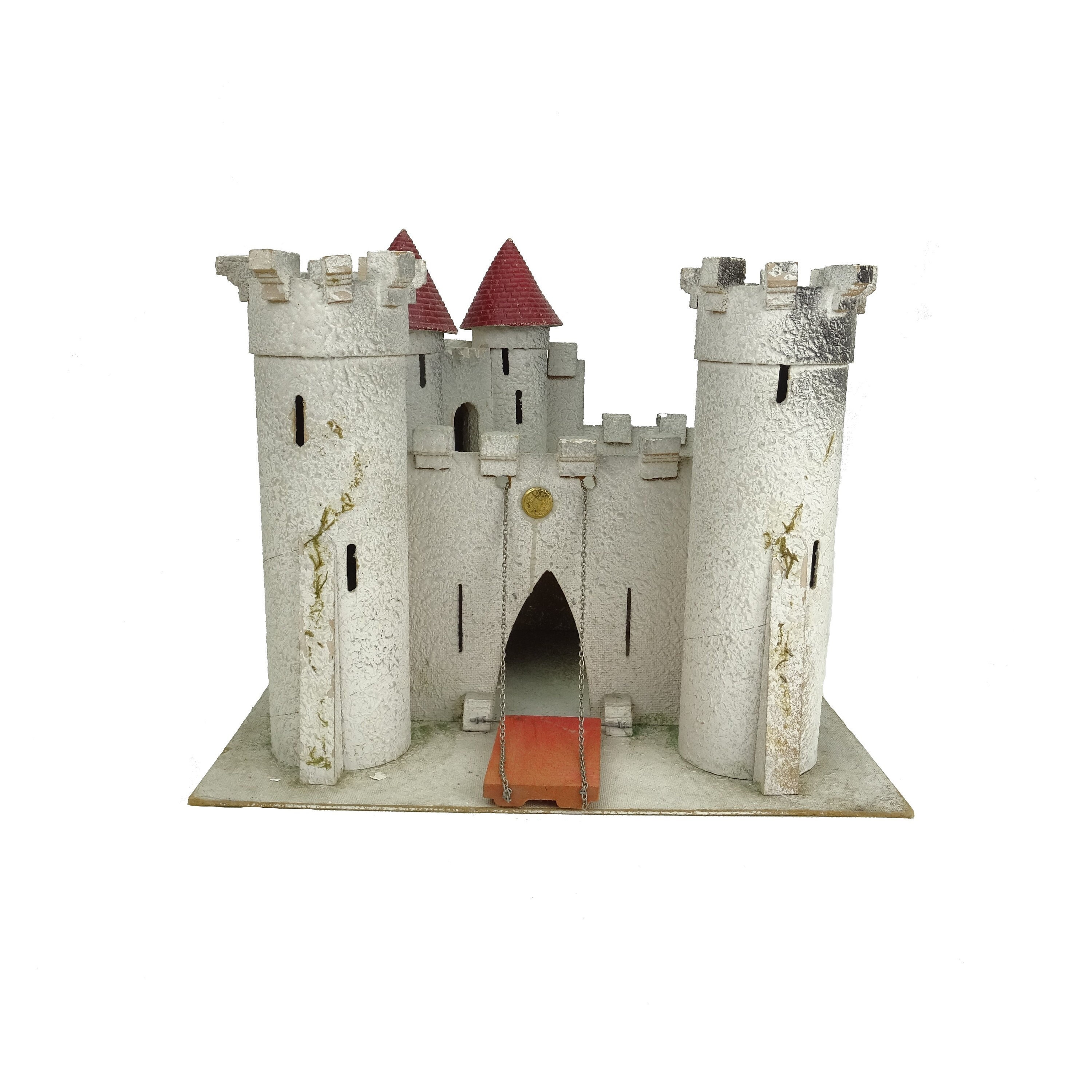The image depicts a highly detailed, handmade model of a medieval castle, set prominently against a completely white background. The castle is predominantly white, with touches of rusty white and black shading that lend it an aged, weathered appearance. The structure features a large, central arched gate with a red, chain-hung drawbridge. There are two large cylindrical front towers with square battlements, each adorned with patches of green moss. The right tower has a slightly blackened top, while the left maintains a whiter hue. Behind these towers, the castle includes two smaller conical turrets with red, cone-shaped roofs. The model is mounted on a square piece of board, possibly steel or cardboard, suggesting it is crafted from arts and crafts materials. The emphasis on the castle’s intricate architectural elements and the barren background highlights its solitary, historic charm.